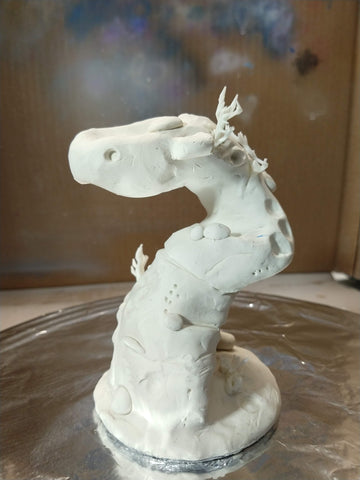The image features a unique white clay sculpture that appears to be an abstract representation inspired by underwater life, resembling a piece of coral or perhaps a seahorse. The sculpted form elegantly zigzags upwards, culminating in a shape reminiscent of a question mark, with a small finger-like extension at the top pointing left. The base of the sculpture is circular, resting on a round sheet of aluminum foil, adding a metallic contrast to the matte white clay. The background is a blurry cardboard box with random paint splotches, enhancing the artwork's raw and creative presentation. This intriguing piece, which might be a school project, combines elements of marine life and mythical creatures, featuring tiny arm-like protrusions and ridges along its twisted neck that evoke a horse-like appearance.